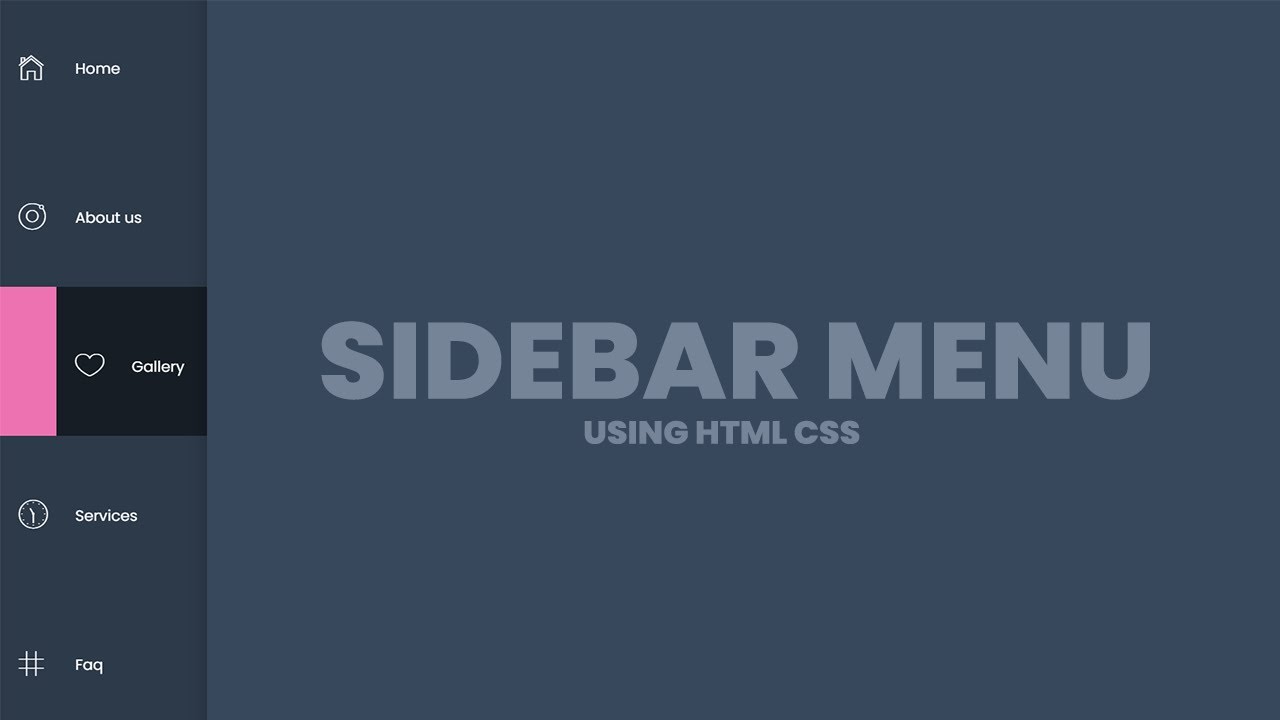This image showcases a sidebar menu designed using HTML and CSS, positioned centrally within the frame against a slightly darker blue-gray background. The sidebar, a light blue-gray rectangular section, features navigational options on the left side, listed vertically. The options include "Home," "About Us," "Gallery," "Services," and "FAQs," with "Gallery" notably highlighted. This highlighted option appears in white text, underscored by a pink line, set against a black background, and accompanied by a white-outlined heart icon.

The title "Sidebar Menu" dominates the image in large, all-capital letters, emphasizing its importance. Below the title, the text "using HTML CSS" appears in a mix of uppercase and lowercase letters. These texts are displayed in white, contrasting with the darker blue-gray sidebar.

The design's color palette includes various shades of blue-gray, white, black, and a touch of pink, creating a clean and visually appealing interface. The image does not provide context as to whether it represents a mobile or tablet view.